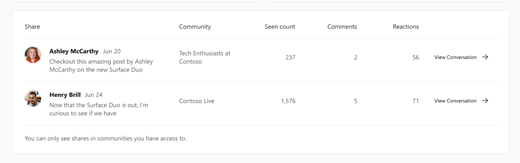This image is a screenshot that appears to be a section of a website or app. The overall shape of the screenshot is a long rectangle, bordered by a narrow gray margin. The predominant background color within the rectangle is white.

At the top of the capture, there are several tabs labeled "Share," "Community," "Scene Count," "Comments," and "Reactions." Below these tabs, the content is divided into individual user instances or profiles.

The first profile is of Ashley McCarthy, a Caucasian middle-aged female. Her profile picture is displayed alongside her name. Her description reads, "Check out this amazing post by Ashley McCarthy on the new Surface Duo." She is identified as a "Tech Enthusiast at Contoso." Her post has a scene count of 237, 2 comments, and 56 reactions. To the right of her profile, there is a button labeled "View Conversation."

The second profile belongs to Henry Brill, identified as a male. His post says, "Now that the Surface Duo is out, I'm curious to see if we have." He is affiliated with the "Contoso Live" community. His post has a scene count of 1,576, 5 comments, and 71 reactions. Another "View Conversation" button is situated to the right of his profile.

At the bottom of the screenshot, there is a note stating, "You can only see shares in communities you have access to."

Overall, the image captures a detailed view of user interactions and posts within a tech-focused community, highlighting individual contributions and engagement metrics.